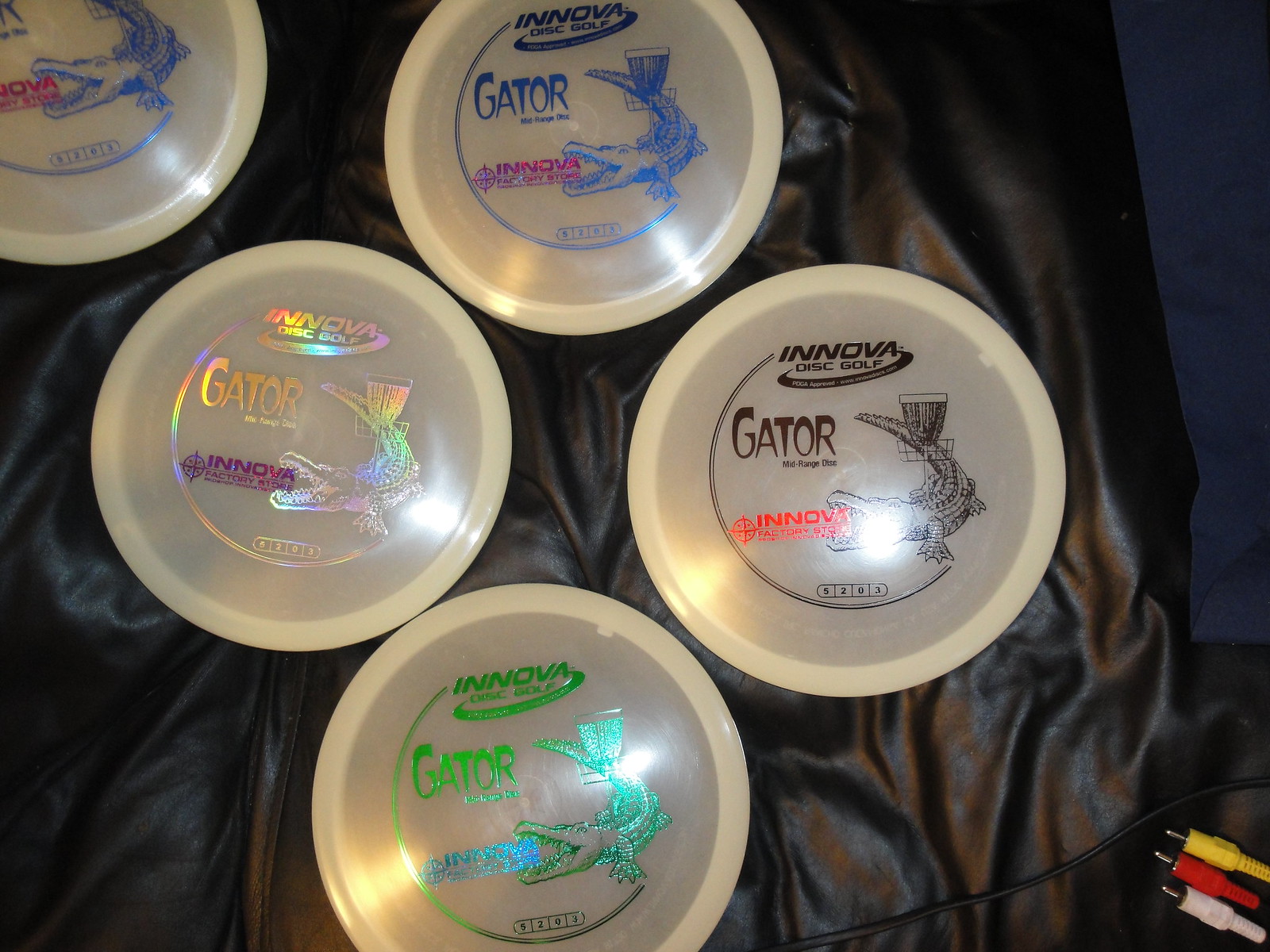This image, taken from above, showcases five plastic Innova Disc Golf Frisbees arrayed against a dark, wavy cloth background, possibly leather. Each disc prominently features a gator graphic wrapped around a disc golf basket with the text "Innova Disc Golf" at the top and "Gator" beneath it. The discs are identical in size but differ in logo and text colors, including combinations such as blue gator with pink writing, an iridescent rainbow-colored gator, green and blue mixed writing, and black or red text. Additionally, some distinguishable features include unreadable four-digit numbers on each disc. In the bottom right corner of the image, several audio-video cables (white, red, and yellow) are visible, hinting at the context of a living room or media setup.